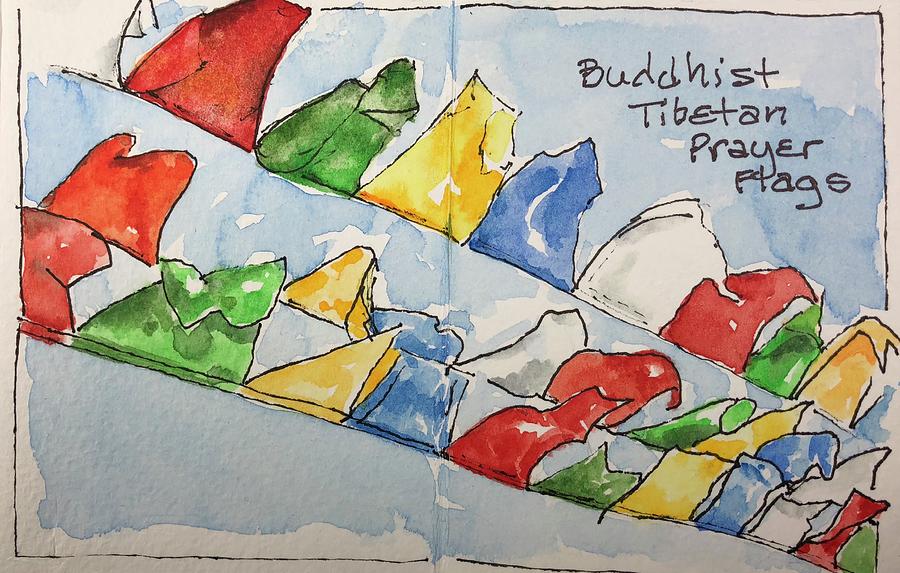This piece of artwork is a detailed watercolor painting that depicts a serene blue sky as its background. Positioned diagonally from the upper left to the lower right are three rows of Buddhist Tibetan Prayer Flags. These triangular flags, reminiscent of colorful tents, are connected along strings that create a striking visual pattern. The flags follow a repetitive color sequence: white, red, green, yellow, and blue. In the topmost row, the sequence is white, red, green, yellow, blue, while the bottom two rows are organized in alternating patterns, with one row starting in red and another beginning in white. The upper right corner of the painting features black text that clearly reads "Buddhist Tibetan Prayer Flags," lending context to the scene. The overall effect is that of a peaceful, cascading line of prayer flags against the calming expanse of the sky.